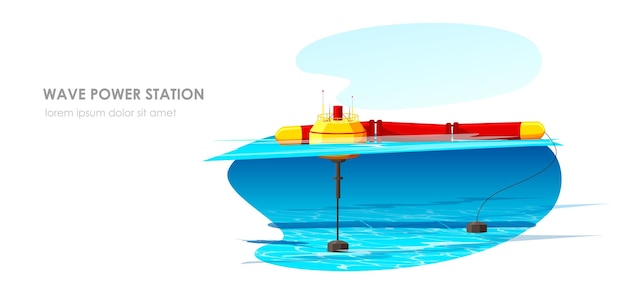This image appears to be an informational diagram of a wave power station, represented as a detailed computer-generated model. The station, predominantly colored in yellow and orange, is shown anchored in a body of water. The structure features an anchor at the rear, securing it to the sea floor, as well as another apparatus extending downward, possibly resembling a drill. Below the image, there is placeholder text written in Latin, "Lorem ipsum dolor sit amet," which is commonly used in design to indicate where text will eventually be placed.